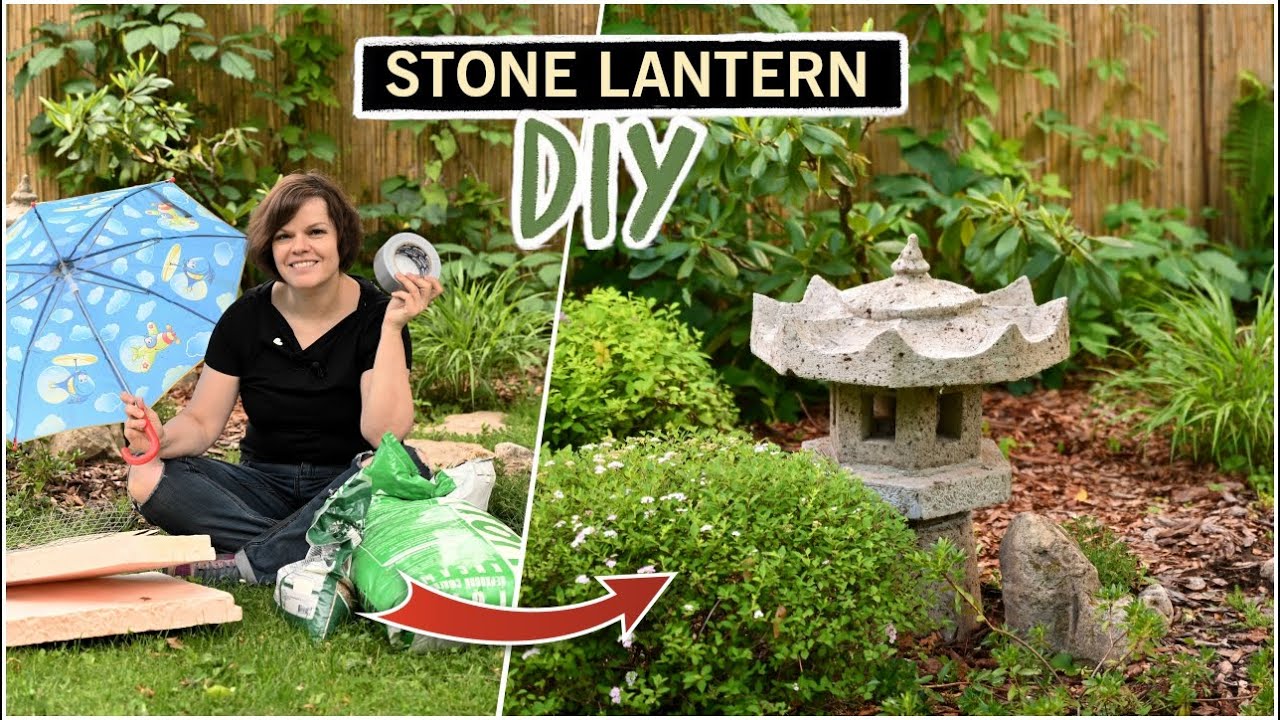The image appears to be a professional advertisement—or possibly a YouTube thumbnail or website banner—promoting a do-it-yourself stone lantern project. On the left side of the diagonally split image, a woman with short dark hair, dressed in a black shirt and pants with a hole at the knee, is seated in her yard. She holds an umbrella in one hand and a roll of duct tape in the other, surrounded by materials needed for the project, including a green bag which likely contains cement. Behind her is an array of plants, adding a lush backdrop. In front of her to the right lies a peach-colored slab. On the right side of the image, the same space is shown post-transformation, depicting a beautifully constructed stone lantern that resembles a pagoda, surrounded by greenery, wood chips, and ornate bushes set against a wooden fence. A red arrow points from the left to the right side, highlighting the transformation process. Above, a black text box with tan letters reads "Stone Lantern DIY." The overall photo quality is high, with vivid colors, excellent lighting, and strong contrast, making the instructional image visually striking and professional.